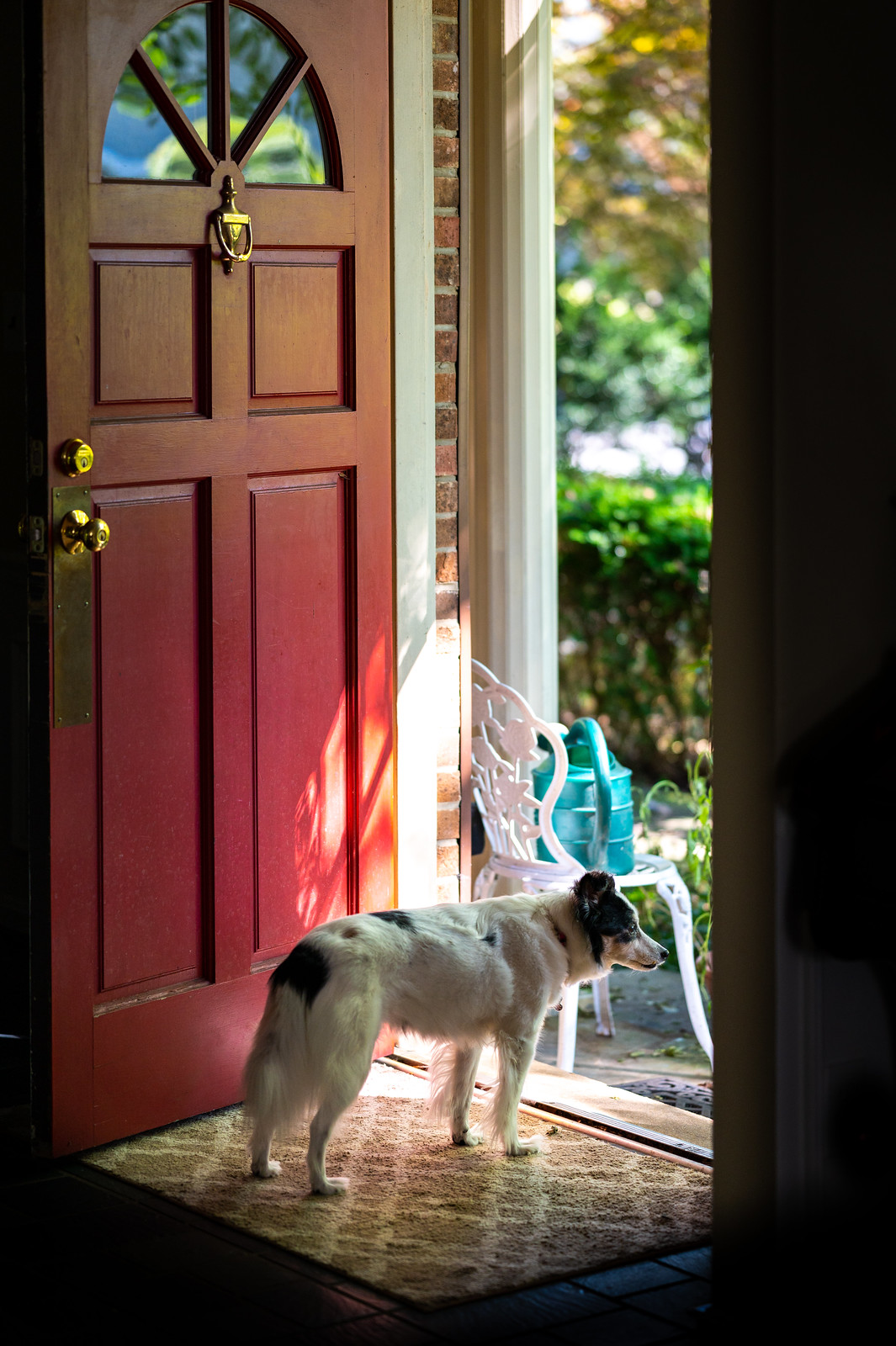In this detailed image, a white and black long-haired dog sits in an open doorway of a red brick house, attentively looking outside. The dog has distinctive markings, with black at the base of its tail, on its right eye and ear, while the rest of its body is predominantly white. The door itself is striking, painted red with a gold or brass door knocker, matching doorknob, lock, and a small decorative brass rectangle beneath the doorknob. The upper part of the door features four pie slice-shaped glass panels forming an arch. Inside the entryway, the dog rests on a tan and white carpet. Outside, the scene is illuminated by sunlight, showcasing a brown doormat and vibrant garden elements. To the left of the door, there is a white chair with a green watering can placed on top. Further out, green shrubs with deciduous trees sporting a blend of green and orange leaves complement a white pillar that is part of the house's foundation. The image captures a serene daytime setting with architectural and natural elements harmoniously presented.